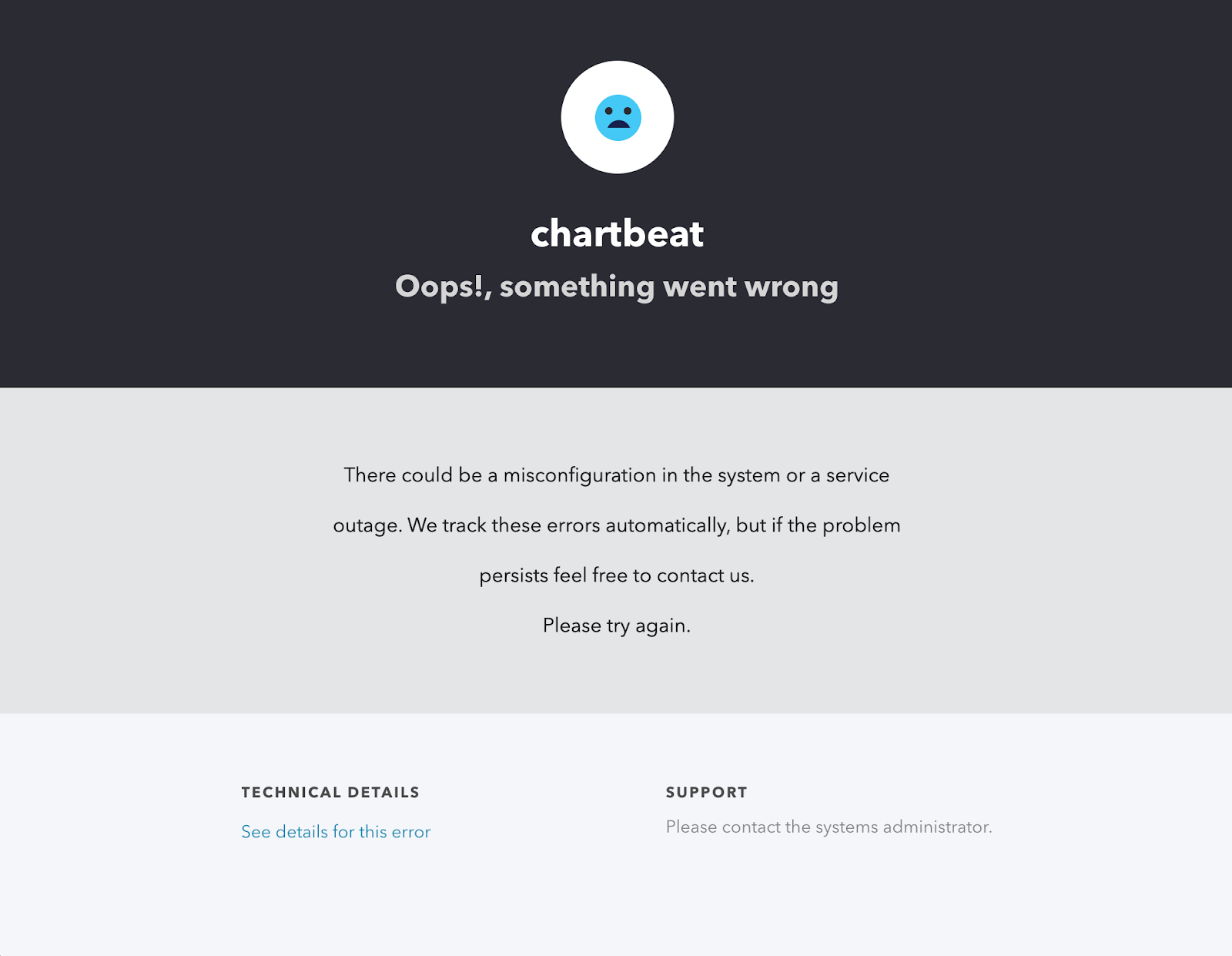A screenshot of an error screen prominently displaying a three-section webpage often seen on product websites or help portals. 

**Top Section:**
- The background is black, with a central logo featuring a white circle, enclosing a smaller blue circle with a face.
- Below the logo, the text "Chartbeat" appears in bold white letters, followed by the message "Oops, something went wrong" in bold gray letters.

**Middle Section:**
- The background is gray, with a centrally-aligned block of small sans-serif text.
- The text reads:
  - "There could be a misconfiguration in the system or a service."
  - "Outage."
  - "We track these errors automatically, but if the problem persists, feel free to contact us."
  - "Please try again."

**Bottom Section:**
- The background transitions to a very light gray, nearly white color.
- This section features the following text:
  - "Technical details: See details for this error" in a blue hyperlink.
  - To the right, it states, "Support: Please contact the systems administrator."